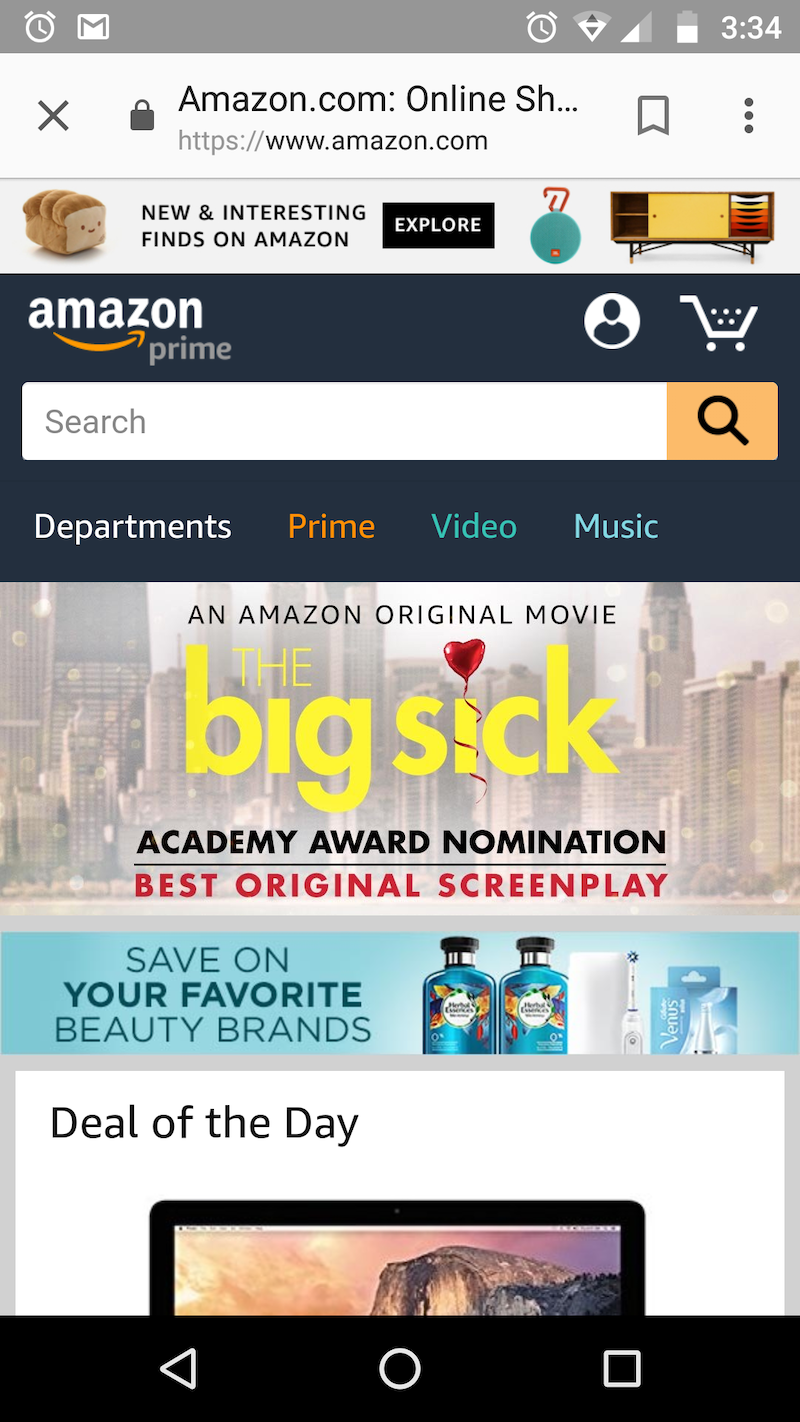On a smartphone screen, the Amazon Prime app is displayed prominently. At the top left, one can see a white clock and the Gmail logo. On the top right, there's another clock, multiple Wi-Fi signal icons with arrows pointing up and down, and a battery life indicator. The time displayed is 3:34 PM. Below this, there is an X icon with a lock beside it, and the text "amazon.com Online Shopping" appears. A bookmark icon and three dots are positioned nearby.

Beneath this, a banner showcases the text "New and Interesting Finds on Amazon" accompanied by a smiley face with a slice, stating "It's got bread." There’s an "Explore" button along with various images, including an ornament with a red hook, some entertainment-related items, and a retro-looking shelf.

A dark navy banner below this reads "Amazon Prime," with "Amazon" in white and the iconic orange swoosh beneath it. To the right on the banner, there's a white shopping cart icon and a user icon indicating where to sign in.

Further down, a search bar with a magnifying glass icon prompts users to type and search for desired items. Below the search bar, there are different tabs: "Departments" in white, "Prime" in orange, "Video" in blue/teal, and "Music" in white/blue.

Prominent advertisements include a highlight for the original movie "The Big Sick," which boasts an Academy Award nomination for Best Original Screenplay. Additionally, there's an ad for beauty brands featuring toothpaste and Herbal Essences products. Lastly, there's a "Deal of the Day" section, displaying an image of an iPad against a mountain backdrop.